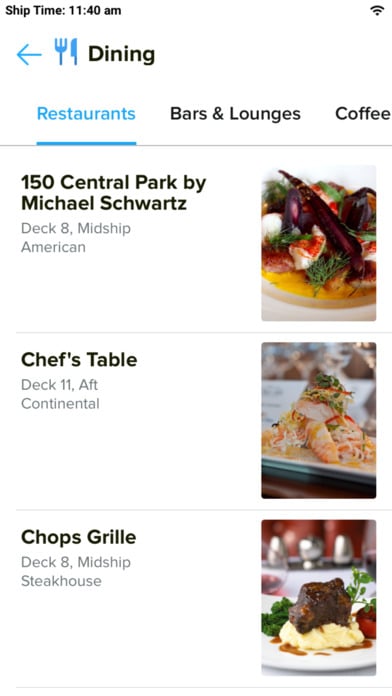The image appears to be a digital interface displaying dining options on a cruise ship. At the top of the screen is "150 Central Park by Michael Schwartz," located on Deck 8, midship, offering American cuisine. The accompanying picture showcases a vividly colored dish with a bright yellow sauce and a garnish resembling a fin, though the exact contents of the dish are indeterminate.

The second restaurant listed is "Chef's Table," situated on Deck 11, aft, serving continental cuisine. The image for this option depicts an intricately decorated dish resembling a starfish with a cat's head, suggesting an artistic culinary presentation, though it is likely an abstract gourmet dish.

The third dining option is "Chop's Grill," spelled with a 'g-i-l-l-e,' also on Deck 8, midship, specializing in steakhouse fare. The picture for Chop's Grill features a thick cut of fillet steak, garnished with grilled tomatoes, served atop a bed of mashed potatoes, and accompanied by a green vegetable, possibly asparagus.